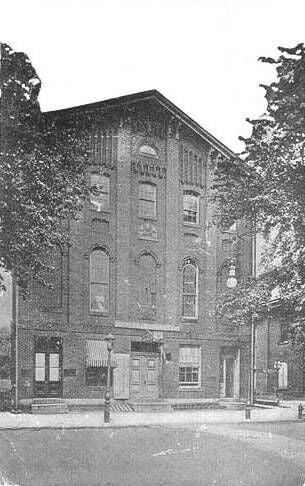This black and white photograph showcases an old, four-story building that exudes an aura of historical significance, suggesting it might be part of a church or a college campus. The building, captured from what seems like a road or parking lot, features a peaked roof on the upper left side and another symmetrical peak in the center on the right-hand side, creating a visually striking architectural silhouette. Tall, arched windows punctuate the stone facade, which is further adorned with intricate engravings and artwork. Street lamps are positioned in front of this imposing structure, highlighting its grandeur. Flanking the building on both sides are partially visible trees, their leaves providing a natural frame to the scene. At the bottom of the photograph, wooden doors can be seen—one on the left, one in the center, and another on the right—providing entry into what could be a school or religious center. The photograph, timelessly captured in shades of black and white, leaves the sky a blank canvas, suggesting a bright day.